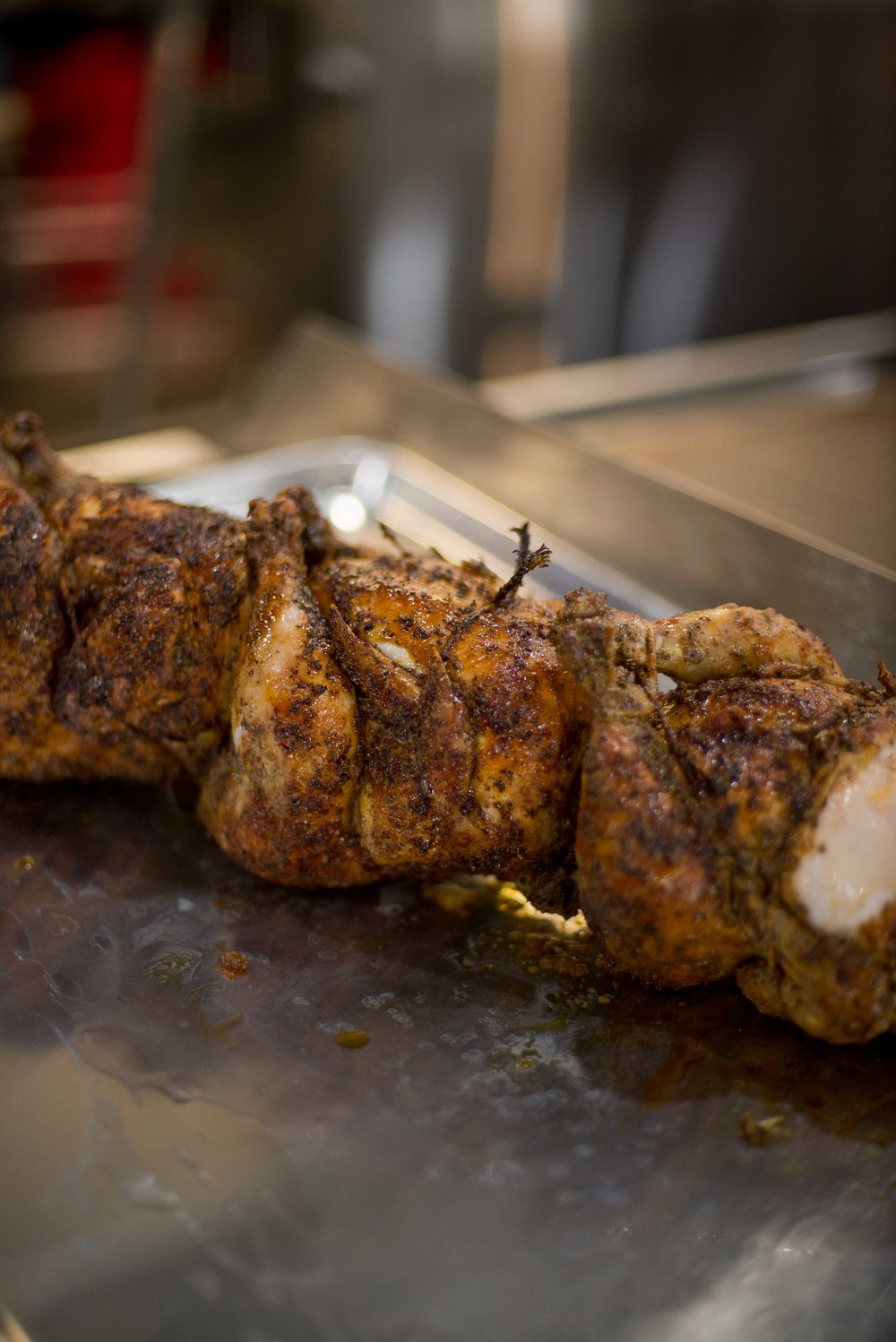The photograph, taken in portrait mode, vividly captures three small, fully cooked birds, possibly rotisserie chickens or Cornish game hens, meticulously arranged in a row on a large metal baking sheet. Their golden-brown, crispy skins are richly seasoned and sprinkled with various herbs, giving them a dark, flaky appearance. Each bird is secured with cooking twine, possibly suggesting they were prepared on an invisible skewer. The baking sheet beneath them glistens with delectable fat drippings, adding to the appetizing presentation. In the background, the image blurs into an indistinct yet unmistakable commercial kitchen scene, featuring stainless steel countertops and appliances. The overall composition highlights the detailed, mouth-watering presentation of the birds while subtly hinting at the professional kitchen environment.